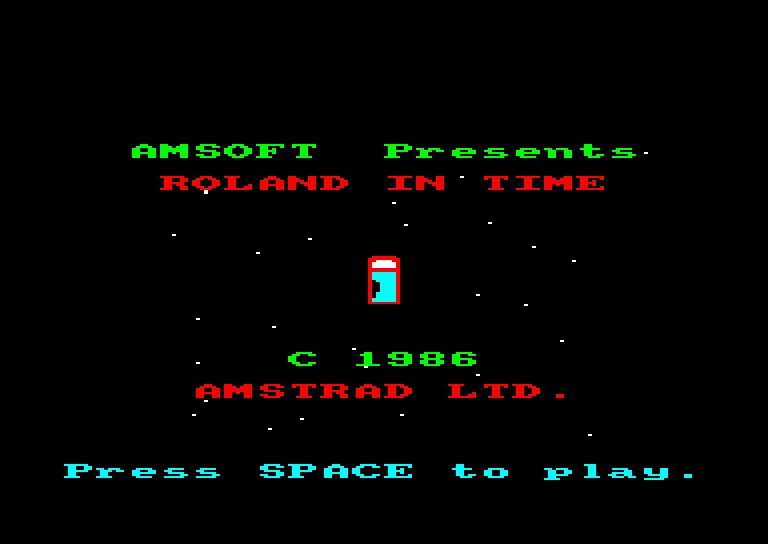The image is a vintage video game screenshot featuring a dark black background with digitized text in a classic 80s video game style. At the top, in bright green letters, it reads "AMSOFT Presents." Below that, in red letters, is the title "Roland in Time." The background displays a starry, space-like graphic with white stars scattered across it. Underneath the title, in green, appears the text "C1986," indicating the year, followed by "Amstrad Limited" in red. At the bottom of the screen, a prompt in bright but light blue letters reads "Press SPACE to play," suggesting that this screenshot is from an early computer game, likely played on an Amstrad system from the mid-1980s.